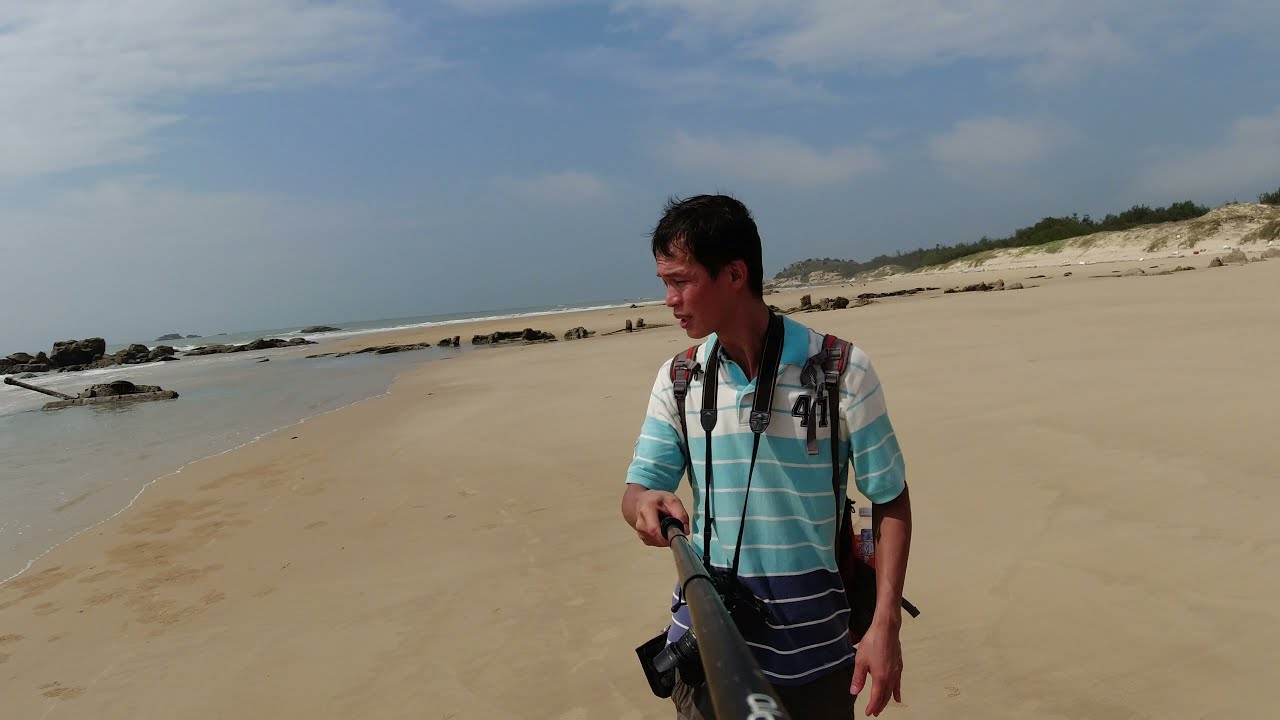In the image, a dark-skinned Asian man, who appears to be in his late 30s, stands on a beach with a selfie stick in his right hand. He possesses a lean physique and sports black hair with a notably good hairline. He wears a white and blue striped shirt and a backpack, gazing off to the left toward the water. The background features sandy terrain with large black rocks scattered around and a few trees on the top right. On the left, the photo captures the edge of the ocean with water rolling in, and a submerged black tank is partially visible, with its turret pointing away from the man. The sky above is adorned with clouds, painting a scene that includes hues of blue, white, gray, green, tan, and light blue. This photograph, taken in the middle of the day, illustrates a serene and slightly intriguing beach setting.